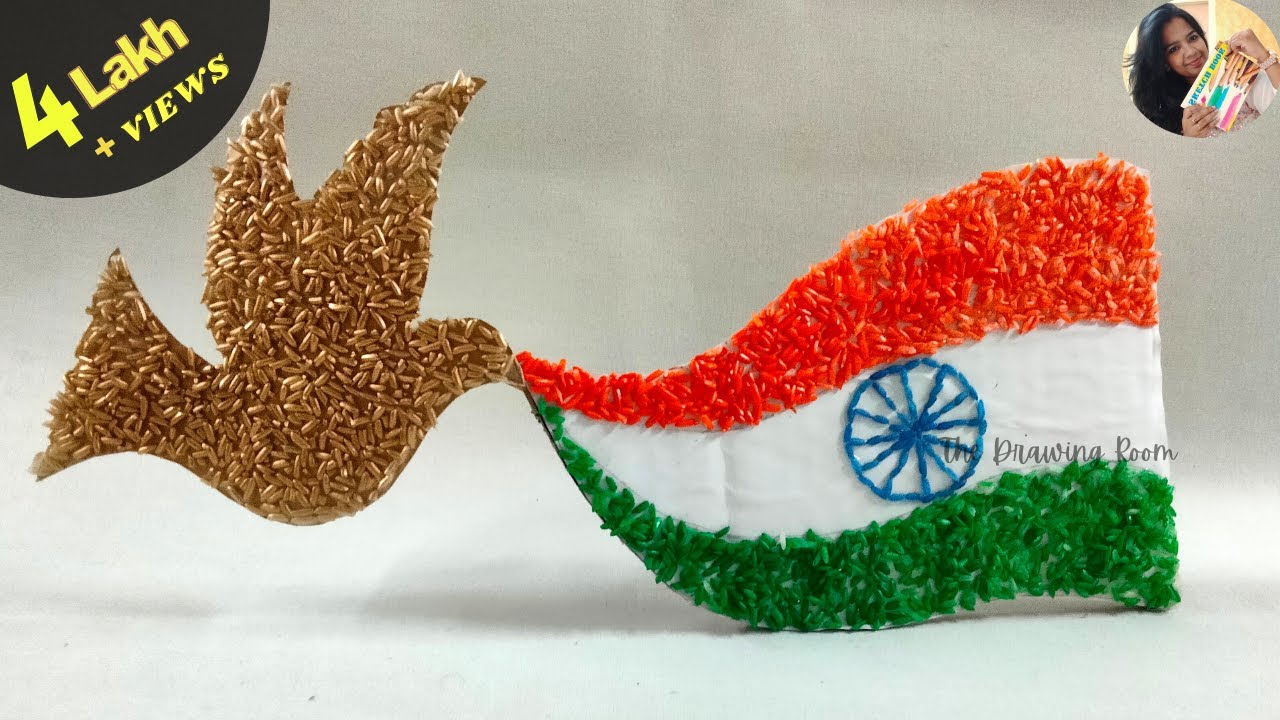This image appears to be a product advertisement or an art piece for sale, featuring a detailed and colorful depiction. Central to the image is a beautifully crafted golden dove with outstretched wings, seemingly made from textured material that closely resembles either sprinkles or small plastic pieces. The dove is holding an Indian flag, characterized by its vibrant orange, white, and green stripes, with a blue wheel in the center of the white stripe. The white stripe of the flag bears the text "The Drawing Room." The background is a clean white box, which emphasizes the colors and details of the art piece.

In the top left corner of the image, there's a prominent graphic featuring a half black circle with yellow lettering that reads "4 Lakh+ views," indicating substantial attention. Additionally, there is a small round photo of a woman in her mid-20s with long black hair holding what appears to be coloring pencils or a pamphlet, slightly tilted to the side. The rich and varied colors within the image include tan, black, yellow, green, red, white, and blue, creating a vibrant and engaging visual.